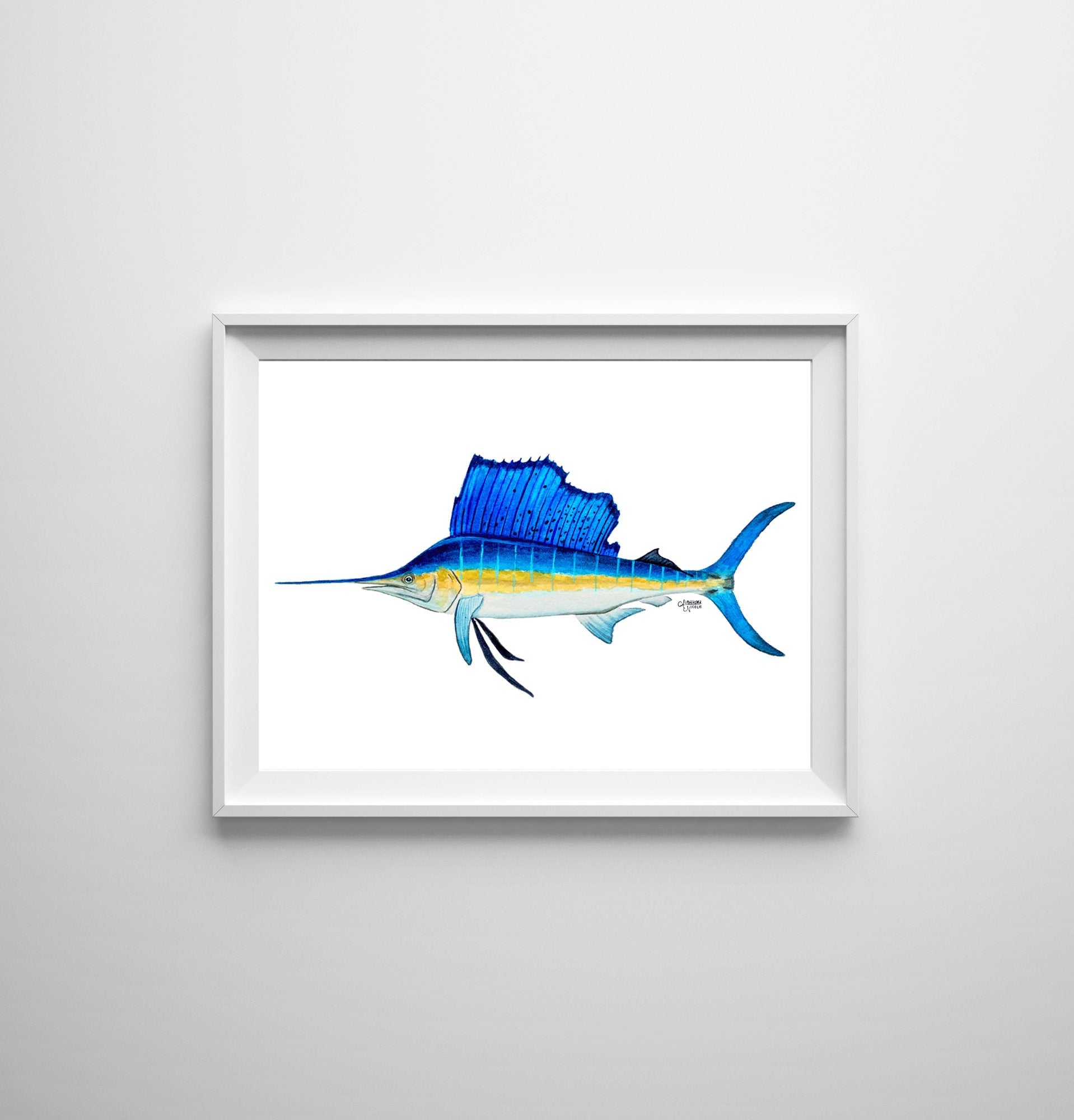This is an image of a blue marlin showcased on a white background, presented within a white frame that's set against a white wall. The marlin, facing left, is depicted in 2D, revealing a detailed left profile. Its top side is painted a rich cerulean blue, transitioning to slightly lighter blue shades towards the lower parts. The marlin's dorsal fin and tail are also blue, with darker blue hues towards the tail's rear. A sharp, needle-like nose extends prominently in a blue tint. The fins on the sides and underneath the marlin exhibit a gradient from light blue to white. Its underbelly features a very light gray color, bordered by a striking golden stripe along its midsection. There is a small black signature visible on the image, though it is too tiny to be deciphered. The overall setting hints at overhead lighting, as indicated by the slightly darker shade at the bottom of the wall.